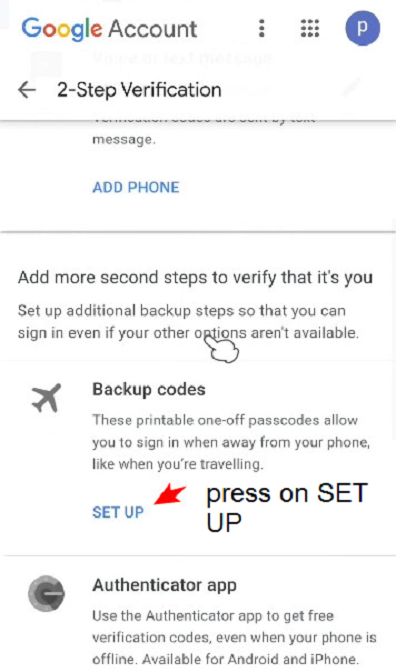A vertical image presumably captured from a mobile device displaying a Google Account webpage. The background is predominantly white. At the top of the page, the header "Google Account" is visible, accompanied by an icon of three vertical dots to its right, followed by a grid icon of nine dots, and a circular avatar with the letter "P" inside it.

Below the header, the section titled "Two-step verification" is prominently displayed, with a left-pointing arrow indicating a navigational option to go back. Under this heading, the text "ADD PHONE" appears in bold blue capital letters. Further down, the page provides guidance for enhancing account security with additional second steps for identity verification.

The instructions explain the setup of backup codes, described as printable one-time passcodes that enable account access when the user is away from home. A "Setup" option is provided for users to configure these codes. Additionally, the page explains the benefits of using an authenticator app for account security. The description highlights that an authenticator app can generate verification codes even when the phone is offline, and specifies availability for both Android and iPhone devices.